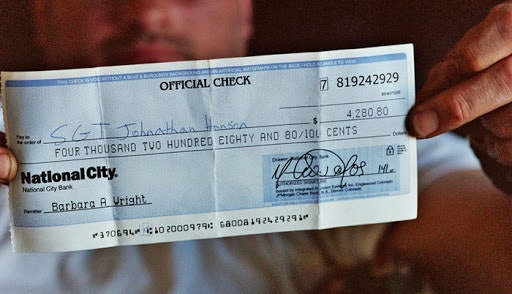In this close-up image, a man wearing a white t-shirt and sporting a black mustache is holding an official check from the National City Bank. The check, which is blue in color, is made out to SGT (spelled S-G-T) Jonathan Hansen, though part of the last name is obscured by a folded crease. The check is for the amount of $4,280.80, with the amount printed both numerically and in words. The handwritten name "SGT Jonathan Hansen" appears on the check, suggesting it is specifically issued to him. Additionally, the bottom left of the check features the printed name Barbara A. Wright. The check number, 819242929, is clearly visible on the document. The image is detailed enough to show the intricacies of the check, emphasizing its official nature.